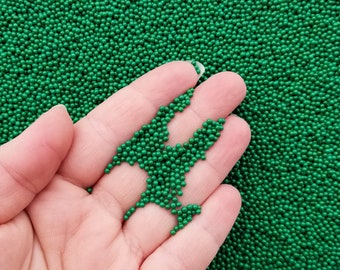The image features a left, light-skinned (Caucasian) hand extending from the bottom left corner towards the center, with fingers pointing towards the top right. The hand is palm-up, displaying visible crinkles and dark lines. Surrounding and on top of the hand are numerous tiny, dark green beads that resemble seed beads without holes. These beads are scattered all around, from the space between the ring finger and the pinky down to the palm, and between the fingers up to the tips. The beads are concentrated on the index finger, particularly around the fingernail, and a few are positioned on the thumbnail. The background is filled entirely with these green beads, evoking a pattern reminiscent of St. Patrick's Day decorations.